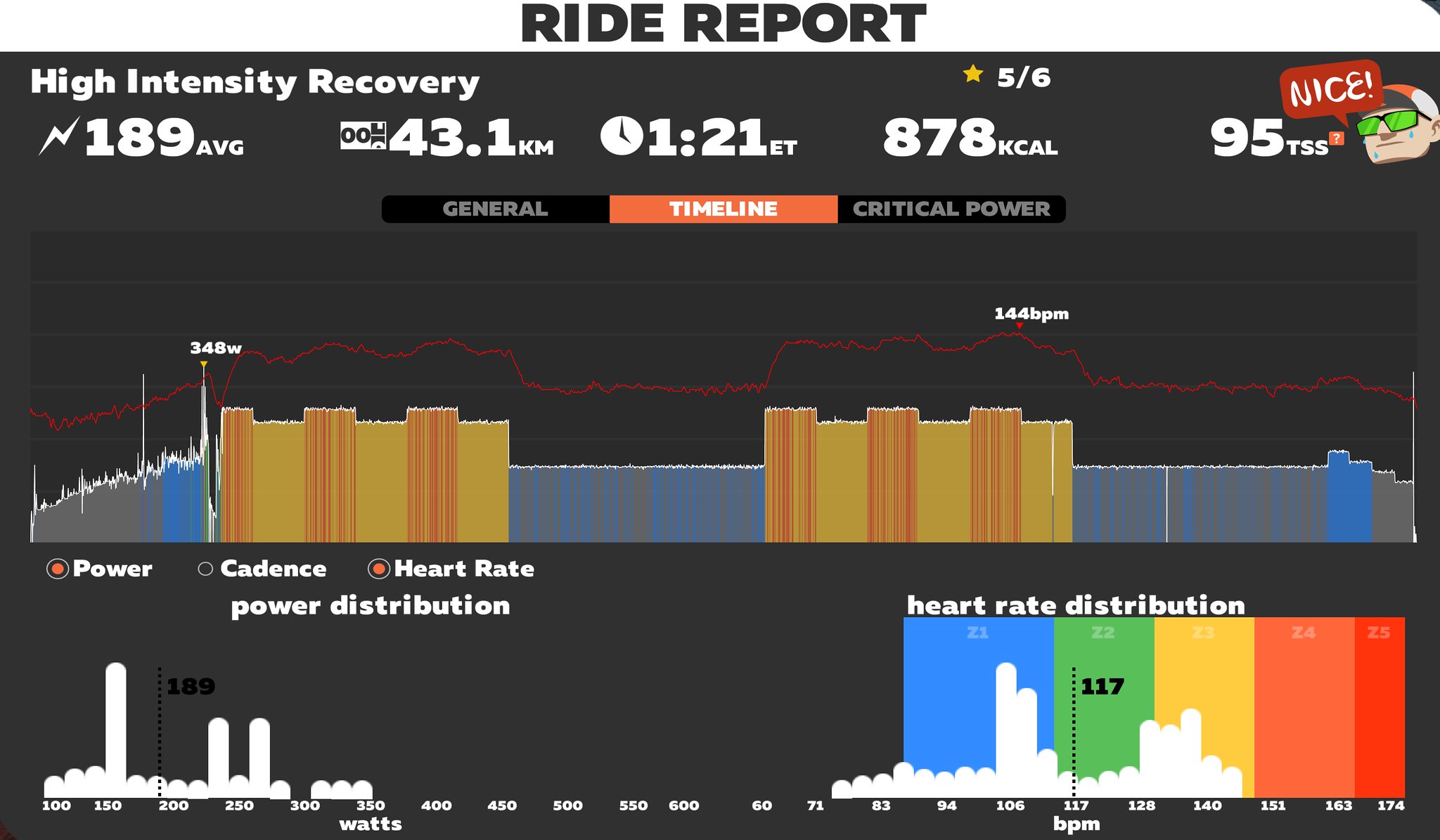This image is a detailed report on a cycling session, rectangular in shape and wider than it is tall. The top features a white header with "Ride Report" prominently displayed in black print. Below, the image has a dark gray background. In the top left corner, the white text reads "High Intensity Recovery," and further to the right is a yellow star labeled "5/6." 

In the central portion, starting from the left, there is a white lightning bolt icon followed by the text "189 average." Moving right, the data continues displaying "43.1 KM," "1:21 Eastern Time," "878 calories," and "95 TSS." The upper right corner includes an image of a Caucasian man's head wearing green sunglasses and a hat, with a red speech bubble that says, "Nice."

The next section features tabs labeled "General," "Timeline" (highlighted with an orange background and white text), and "Critical Power," each in black with gray print. Below these tabs are various graphs and charts.

Starting from the left, the first graph has a red jagged line traversing the top, with vertical gray, blue, yellow, and orange lines below. Beneath this graph, a red circle is labeled "Power," while adjacent empty red circles are labeled "Cadence" and "Heart Rate Power Distribution."

At the bottom left, another graph labeled "Watts" ranges from 100 to 350, with a black line marking the value at 189. In the lower right corner, another graph is labeled "VPM," with the term "Heart Rate Distribution" above it. A black bar marks the value at 117 beats per minute, with additional ranges noted as "94," "106," and "117 bpm."

This comprehensive visualization likely pertains to a health or fitness application focusing on cycling metrics and performance analytics.